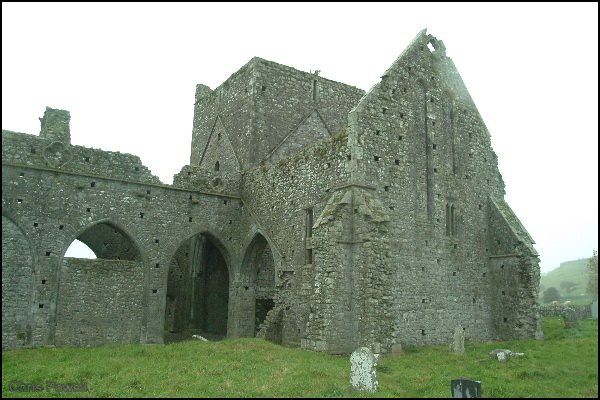The photograph captures the haunting remnants of a centuries-old stone structure, likely a medieval castle or church, situated in an open grassy field. The building, constructed from gray stones, shows significant signs of decay—its roof and arch have collapsed, and parts of the walls are missing, giving it a beleaguered, crumbling appearance. In front of the structure lies a small cemetery with aged tombstones, some chipped and weathered to a grayscale palette over time, including one that hints at having been originally white. A small fence appears in the background, delineating the area. The right side of the scene features a gentle hill dotted with a few trees and bushes. The sky above is a bright, almost blinding white, likely due to a mix of overcast clouds and mist, and a distant hill or a valley looms to the left. Overall, the scene evokes a chilly, misty morning ambiance, amplified by the desolate beauty of the decaying edifice.